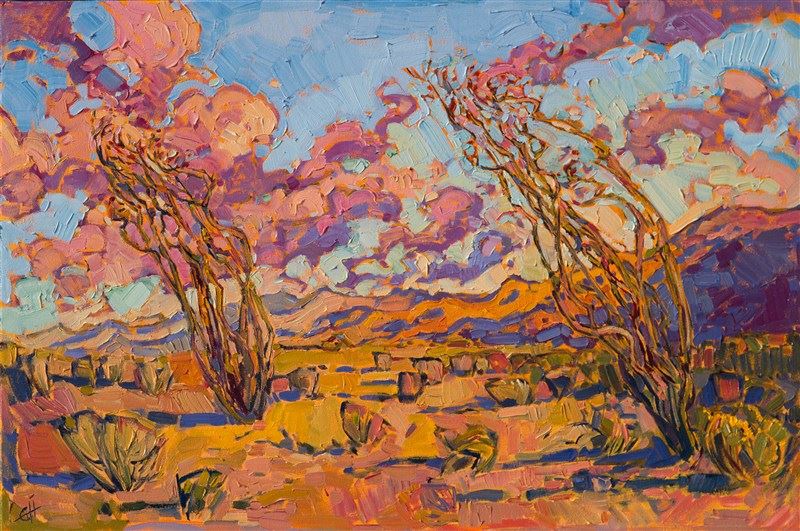The image is a vividly colorful and textured oil painting of a surreal desert landscape beneath a blue sky. The scene features vibrant, wavy clouds in shades of pink, purple, blue, and orange. Stretching across a expansive flat plain that leads to distant, uniquely hued mountain ranges of peach, blue, and dark purple, with golden sunlit areas. The desert ground is filled with small shrub-like plants in green and darker orange hues, and features two tall, thin, nearly leafless plants suggesting aridity. A notable detail is the artist's mark in the bottom left corner, resembling intertwined letters "C" and "H," adding an enigmatic signature to this abstract but comprehensible natural scene.